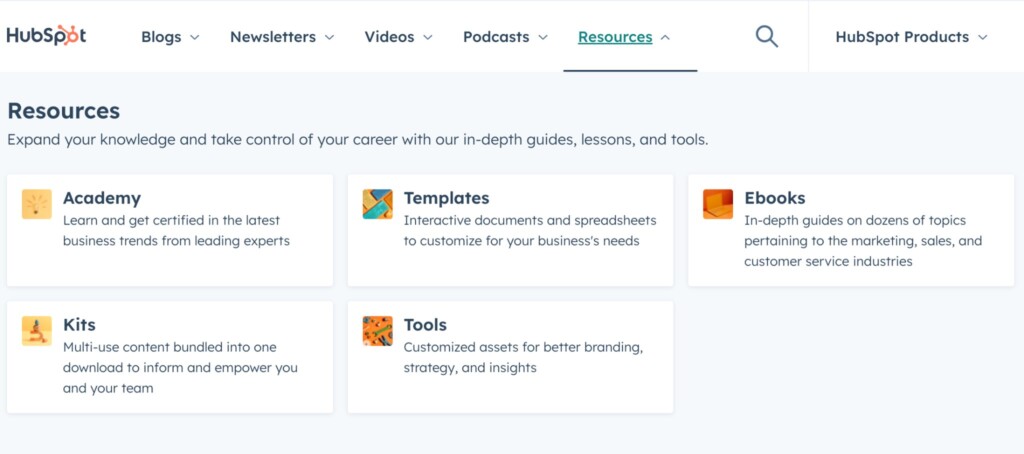This is a detailed caption for an image of a HubSpot screenshot, used as a content management platform.

---

The screenshot displays HubSpot's user interface. In the top left corner, there's the HubSpot logo, which is "HubSpot" in black font, spelled H-U-B, capital S-P-O-T, as one word. The "O" is a distinctive orange color with three little lines extending outwards, ending in small dots. The header background is white.

From left to right in the header, we see navigation options: Blogs, Newsletters, Videos, Podcasts, and Resources. The "Resources" tab is highlighted and underlined in green, indicating the active page. On the right side of the header, there's a search icon followed by the text "HubSpot Products."

Below the header, on the left side, is a main heading that says "Resources" against a very light green background with dark gray font. Beneath this heading, there's a subtitle that reads: "Expand your knowledge and take control of your career with our in-depth guides, lessons, and tools."

The content is organized in white rectangles. In the top row, from left to right, are three categories: Academy, Templates, and eBooks. In the bottom row, there are two categories: Kits and Tools. Next to each category name is a small square icon that varies in color and design. The icon for Academy is light orange, Templates is multi-colored, eBooks is orange, and both Tools and Kits feature multiple colors.

Under each category name, there is a brief description. For example, beneath "Academy," it says: "Learn and get certified in the latest business trends from leading experts."

---

This finalized caption accurately captures the detailed elements and layout of the HubSpot screenshot.